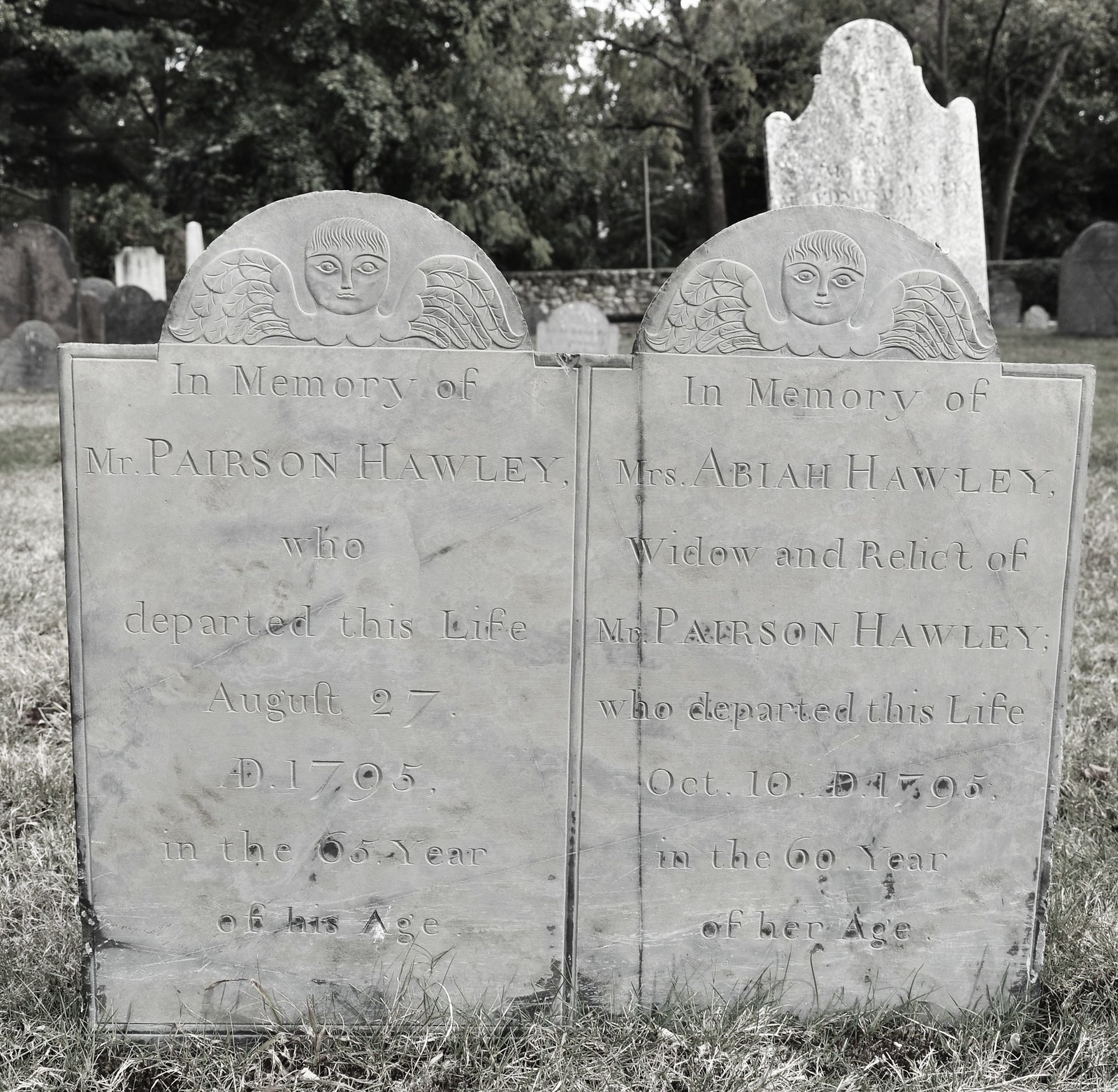This black-and-white photograph captures a serene cemetery scene featuring two slate gravestones set side-by-side in a grassy field. Both gravestones, adorned with carved angels at the top, commemorate the lives of Mr. Parsons Hawley and Mrs. Abadie Hawley, who are likely husband and wife. Mr. Parsons Hawley's gravestone reads, "In memory of Mr. Parsons Hawley, who departed this life on August 27th, 1795." Mrs. Abadie Hawley's gravestone, which specifies her as the "widow and relic of Mr. Parsons Hawley," reads, "In memory of Mrs. Abadie Hawley, who departed this life on October 10th, 1795, in the 60th year of her life." The backdrop consists of more gravestones scattered throughout the grassy field, framed by trees and a stone wall visible in the distance. The dry grass in the foreground adds a touch of timelessness to this poignant image, embodying a peaceful yet somber atmosphere.